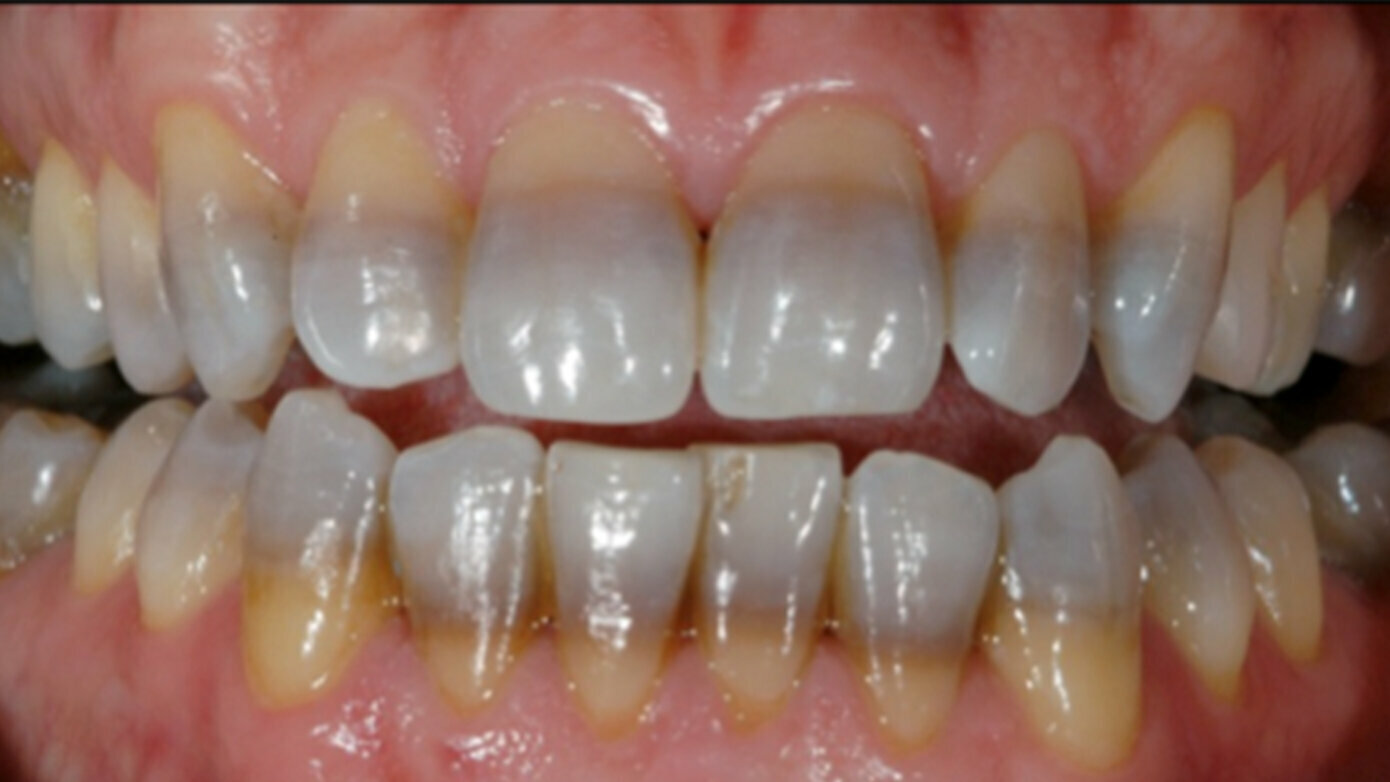This highly detailed close-up image depicts a set of teeth and gums, showcasing dental issues within the mouth. The majority of the teeth are uneven, with the upper teeth appearing white and the lower teeth displaying a notable yellow discoloration. Multiple cavities are evident, particularly on the lower teeth, which have at least three visible cavities, while the upper teeth also show signs but are harder to discern. There's a distinct presence of plaque between the teeth as well.

The gums are a bright pink, framing the teeth in a manner that highlights their irregular condition. A closer inspection reveals a brown line at the base of the teeth, suggesting significant dental problems. The tongue is visible in the background but does not interfere with the focus on the teeth and gums. Despite the dental issues, the teeth have a shiny appearance. The image is a full frontal shot with the teeth nearly touching, emphasizing the front view and the contrasting colors of light pink, pink, light yellow, white, and some black hues. The photograph does not include the lips and provides a comprehensive and unsettling view of the oral health in detail.